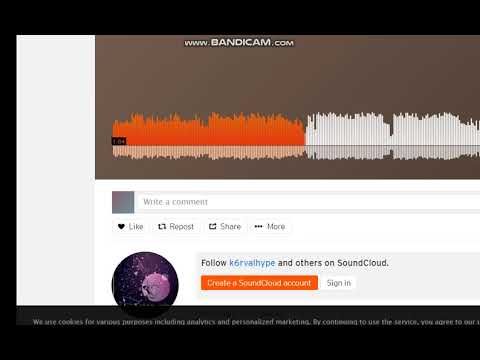The image depicts the left-hand side of a web page from Bandicam (bandicam.com). The page features a predominantly black background with a sectioned layout. The upper portion, colored in chocolate brown, prominently displays "WWW.BANDICAM.COM" in all capital letters. Below this, there is an audio file visualization, starting with an orange waveform transitioning into white.

Beneath the waveform and transitioning into the white section of the page, there is a white comment box where users can write messages. This section includes options to like, repost, share, or access additional features through a "more" option. Continuing downward, a light gray box appears with the message, "Follow K6RVALHYPE and others on SoundCloud,” where the username "K6RVALHYPE" is highlighted in bright blue, and the rest of the text is in gray.

Below this, there is a prominent orange button labeled "Create a SoundCloud account" in white lettering. To the right of this button, there is a smaller gray text button that says "Sign in." To the left of the orange button is an avatar displayed within a circular frame, depicting what seems to be a planet in outer space.